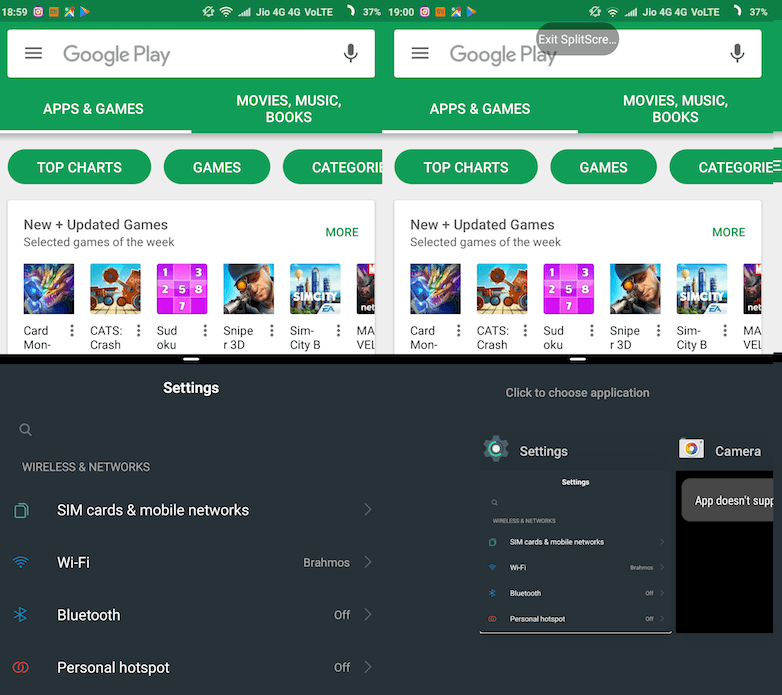A screenshot displays two adjacent instances of the Google Play Store app, each featuring a green bar at the top indicative of Google Play’s interface. This side-by-side arrangement gives an unusual appearance, as if the image consists of two overlapping screenshots. Both Google Play screens exhibit identical features: a 4G VOLTE indicator, a battery level at 37%, and identical tabs offering "Apps & Games," "Movies & Music," "Books," "Top Charts," "Games," "Movies," and "New & Updated Games."

In the bottom section of the image, there is an overlay that seems to merge the two screenshots into one. On the left, the overlay shows a section titled “Settings” under "Wireless and Networks." On the right side of this overlay, another interface is visible, featuring an option labeled "Click to choose the application." This intricate assembly of elements creates a detailed, albeit perplexing, visual of simultaneous interactions within the Google Play Store environment.